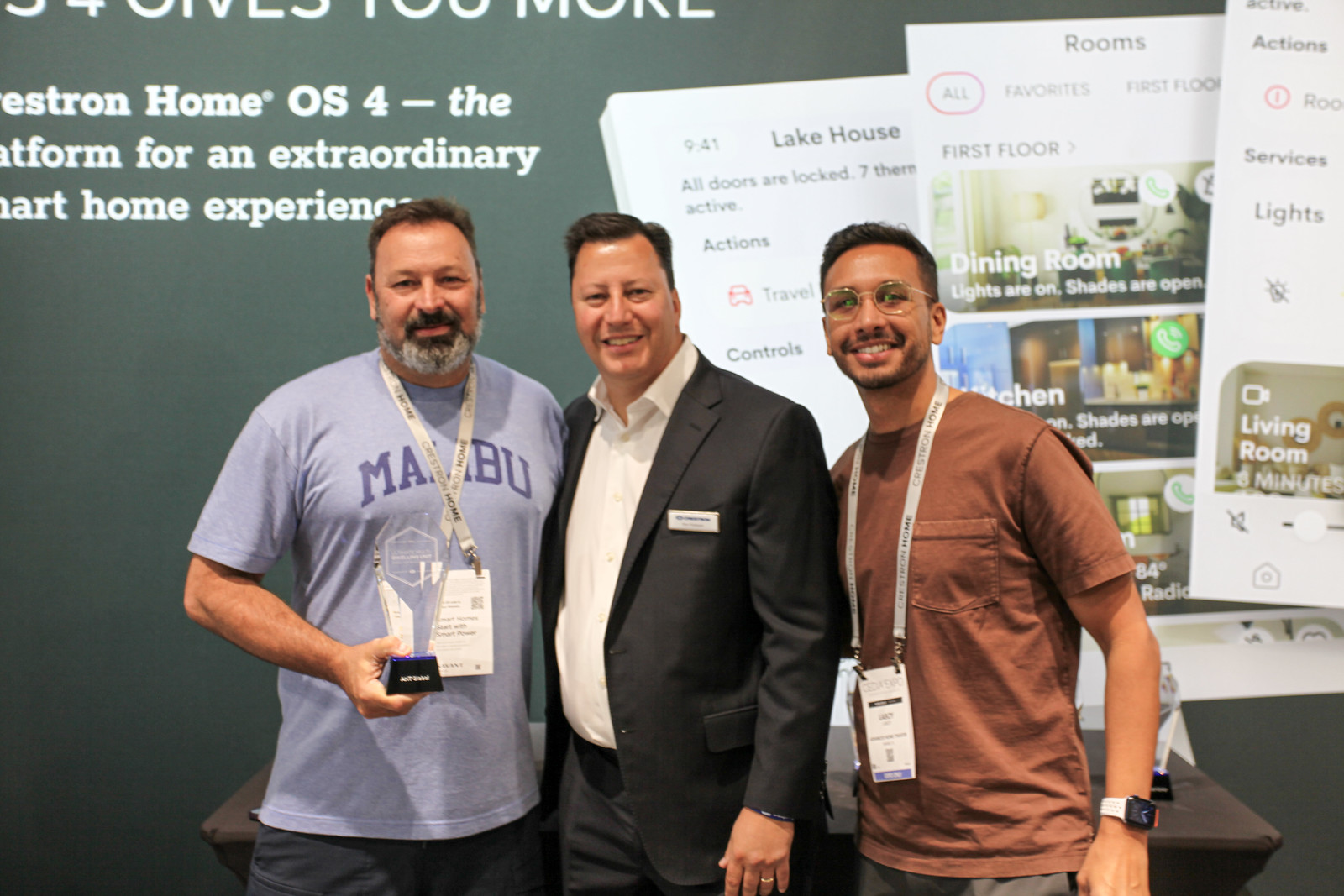In this image, three men are posing in front of a green wall adorned with various signs and brochures related to real estate. The man on the left, who appears to be in his late 40s or early 50s, is holding a crystal trophy with a black base. He is dressed in a blue t-shirt with "Malibu" written on it and gray shorts. He has short brown hair and a salt-and-pepper beard. The man in the middle is wearing a dark gray business suit with an off-white collared shirt and no tie. He has a name tag hanging from his neck. The man on the right is in a rust-colored t-shirt, also with a lanyard displaying his ID, and glasses with gold frames. Behind them, the wall displays text saying "Estrin Home OS4, the platform for an extraordinary smart home experience." To the right are three overlapping brochures that mention "Lake House Rooms," "Actions," "First Floor," and showcase images of a dining room and kitchen, suggesting a real estate or smart home award context.